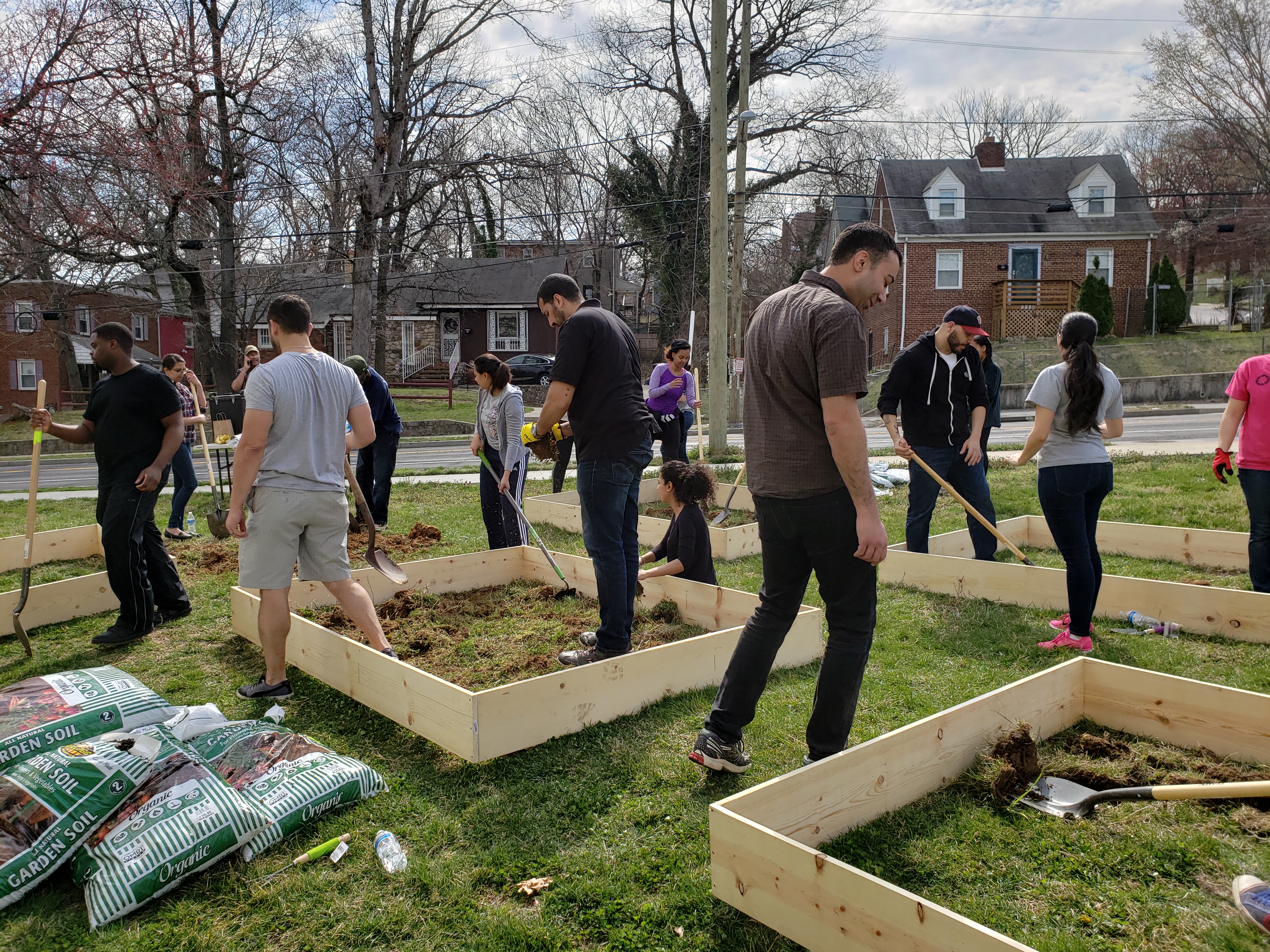In this photo capturing a vibrant community event, a diverse group of individuals—including men, women, and children—are working together to create a community garden in a residential neighborhood. The setting is a plot of green grass surrounded by houses, visible across a nearby street adorned with telephone poles and tall, leafless trees, suggesting it might be fall or early spring. The focal point of the image is the array of rectangular garden enclosures, meticulously constructed from cedar wood planks, likely measuring around 8x12 inches. People are actively engaged in preparing the soil, using shovels, rakes, and hoes. To the left of the frame, bags of organic garden soil, notably in green and white-striped packaging, are piled up, ready for use. Amidst the bustling activity, participants dressed in varied attire—long pants, shorts, and khakis—demonstrate a shared commitment to this communal gardening project.